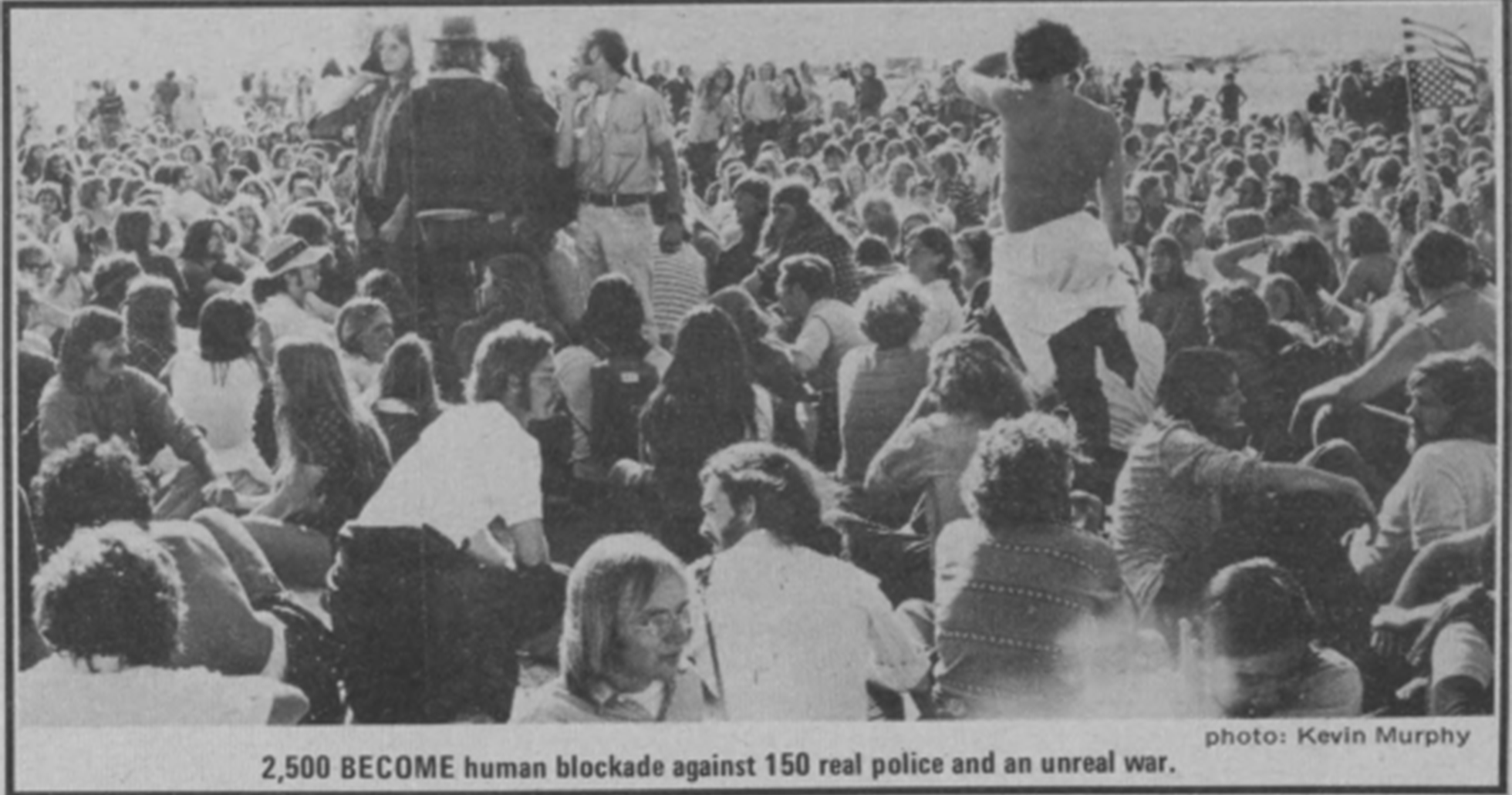This vintage black-and-white photograph, taken by Kevin Murphy and likely from a 1960s newspaper, captures a significant Vietnam War protest. The hazy white background and American flag flying in the upper right corner provide a striking contrast to the somber scene below. A caption beneath the image reads, "2,500 become a human blockade against 150 real police and an unreal war," emphasizing the scale and intensity of the demonstration. The crowd, composed mainly of young people, spans across the frame, with many sitting and some standing, creating rows upon rows of determined faces. Notably, a few individuals with rimless glasses and long hair stand out, while one person in the lower center wears a dark shirt and white pants. On the left, some uniformed policemen can be seen, underscoring the tension of the event. The participants, mostly clad in short-sleeve shirts, suggest the protest took place on a warm summer day.